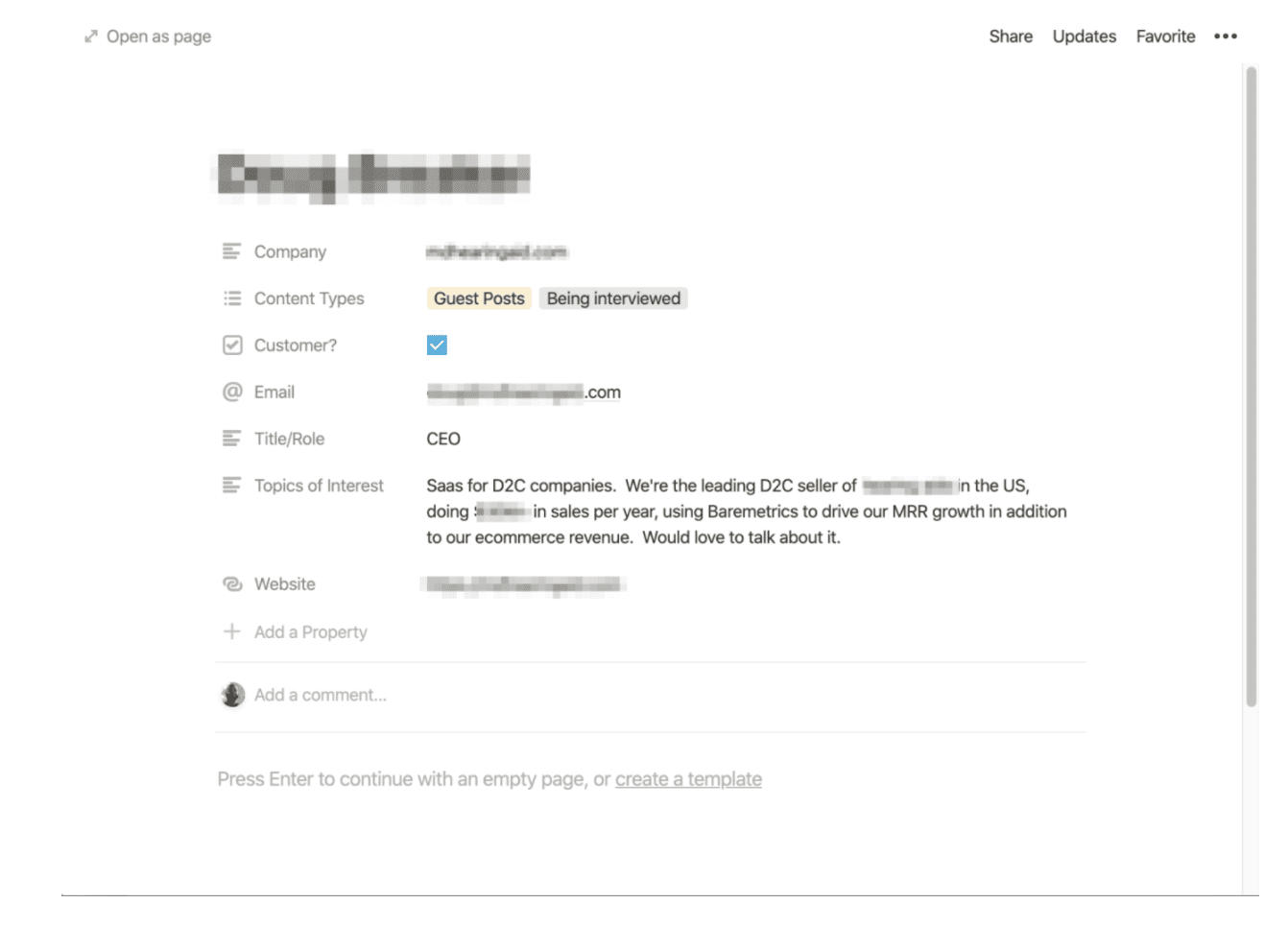This is a detailed screenshot of a web page with a predominantly white background. In the top left corner, the page title reads "Open as Page," while the top right corner features an array of options including "Share," "Updates," "Favorite," and a menu indicated by three vertical dots, all displayed in dark gray. 

At the very top of the screenshot, there is a segment blurred out in shades of gray and white, likely concealing sensitive information.

Below this, the section is labeled "Company," where the company name has also been blurred. The label "Content Types" follows, with two categorizations: "Guest Posts" highlighted with a yellowish background, and "Being Interviewed" marked with a gray background.

Further down, the line labeled "Customer" features a blue box with a white checkmark. The "Email" field is present but the specific email address is blurred, save for the ".com" suffix. The "Title/Role" field is filled in as "CEO."

The text continues with "Topics of Interest," listing "SaaS for D2C companies," and mentioning that the company is a leading D2C seller in the US, though specifics are blurred out. The document notes the use of "Barometrics" to drive MRR growth and indicates significant e-commerce revenue, but specific figures and details are obscured.

The final sections include fields labeled "Website," "Add a Property," and "Add a Comment," which appear unused or intended for further input.